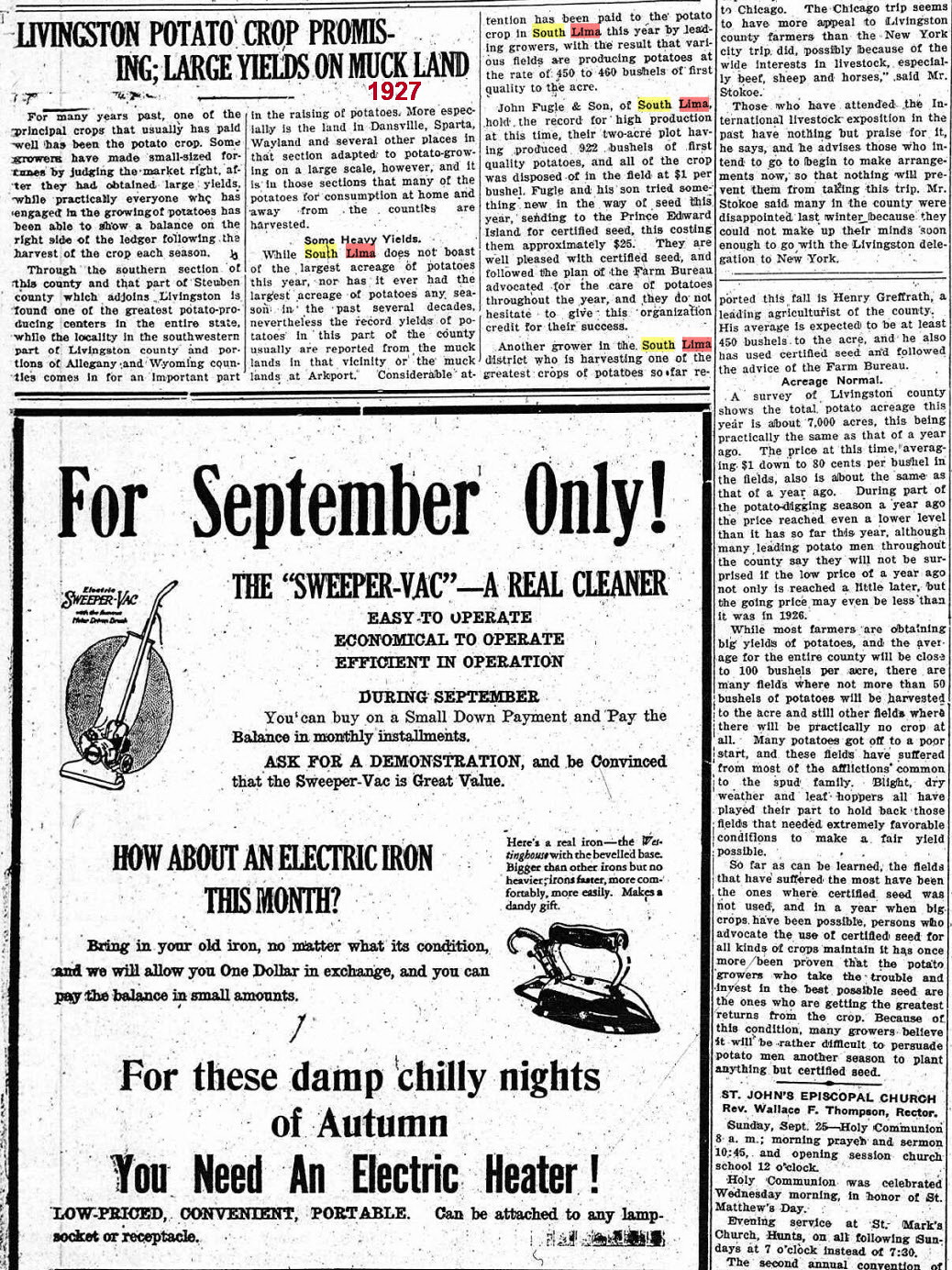The image is a detailed snippet from an old newspaper page dated 1927, featuring an article and a prominent advertisement. The main article, titled “Livingston Potato Crop Promising Large Yields on Muck Land,” is highlighted at the top left with small text spread across the majority of the upper and right-hand portions of the page. Specific words such as "South" and "Lima" are highlighted in yellow and pink respectively within the article.

In the advertisement section, the focus is on several products, starting with a vacuum cleaner highlighted in large letters, “For September Only: The Sweeper Vac, a Real Cleaner.” It describes the vacuum as easy to operate, economical, and efficient, offering a promotion where customers can buy it with a small down payment and pay the balance in monthly installments. The ad encourages customers to ask for a demonstration, ensuring its great value.

Below the vacuum cleaner ad, there is a promotion for an electric iron: “How about an electric iron this month?” It offers a $1 exchange for any old iron, allowing customers to pay the balance in small amounts. A picture of an old-school iron is also part of this section. Lastly, the ad highlights an electric heater suitable for the damp, chilly nights of autumn, emphasizing its low price, convenience, and portability, stating it can be attached to any lamp socket or receptacle.

The overall presentation merges historical context with detailed advertising, capturing both the agricultural news and the household innovations of the time.